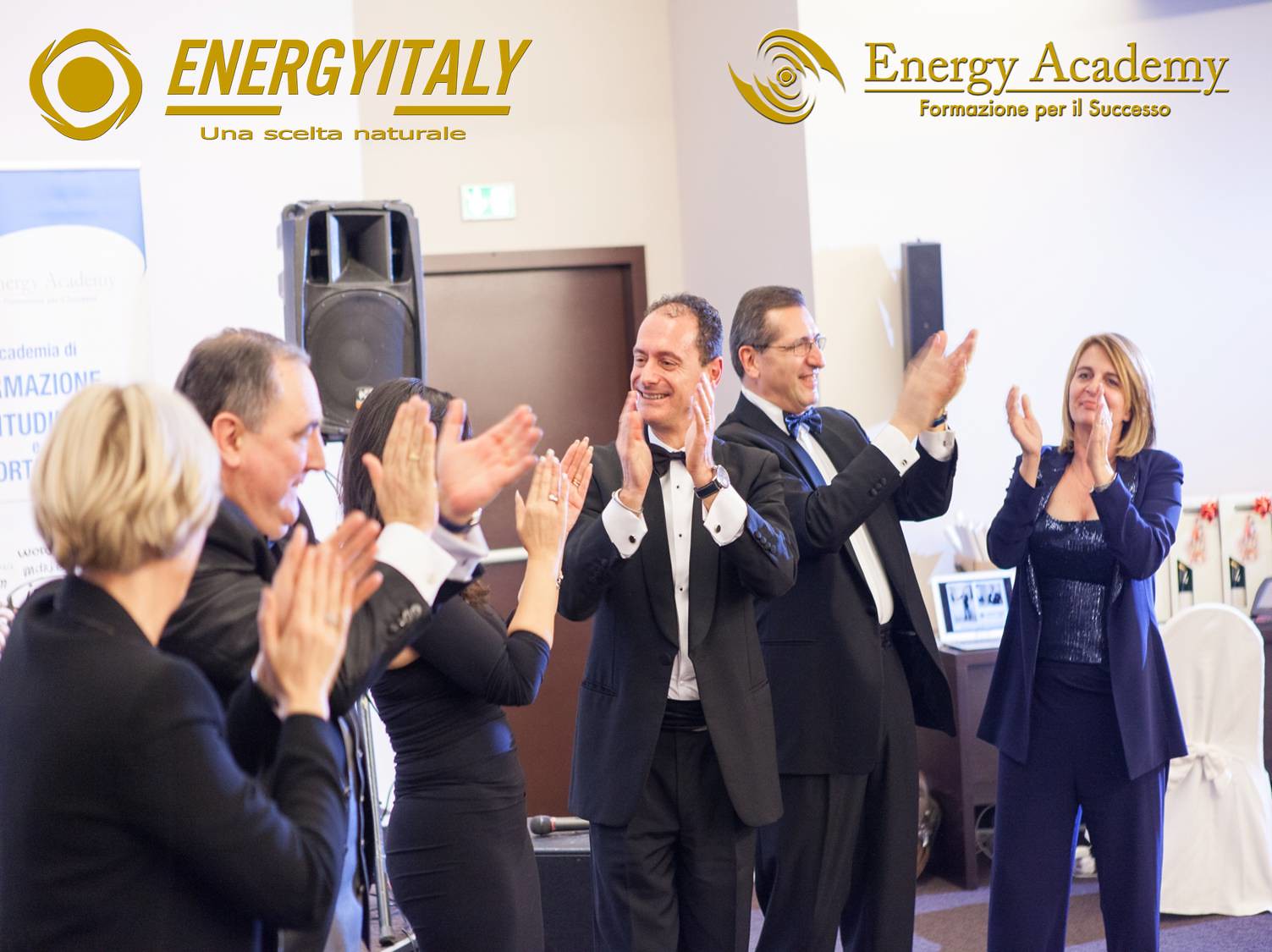In the image, a group of six people, comprising three men and three women, are standing inside a room with white walls and a brown door. They are all dressed in dark suits; the men pair theirs with white shirts, while the women wear dark tops underneath their suits. Everyone is clapping and appears to be in high spirits, with smiles on their faces. Behind them are a desk, a chair, and a speaker on a stand. At the top of the picture, text reads "Energy in Italy" on the left and "Energy Academy" on the right. Each of these titles is accompanied by a distinct logo: the one on the left features a circle with a wavy design, and the one on the right displays a spiral shape. An additional line of text below "Energy in Italy" says "Una Scelta Naturale" in Italian. The consistent theme of energy and enthusiasm is captured as the individuals applaud joyfully.